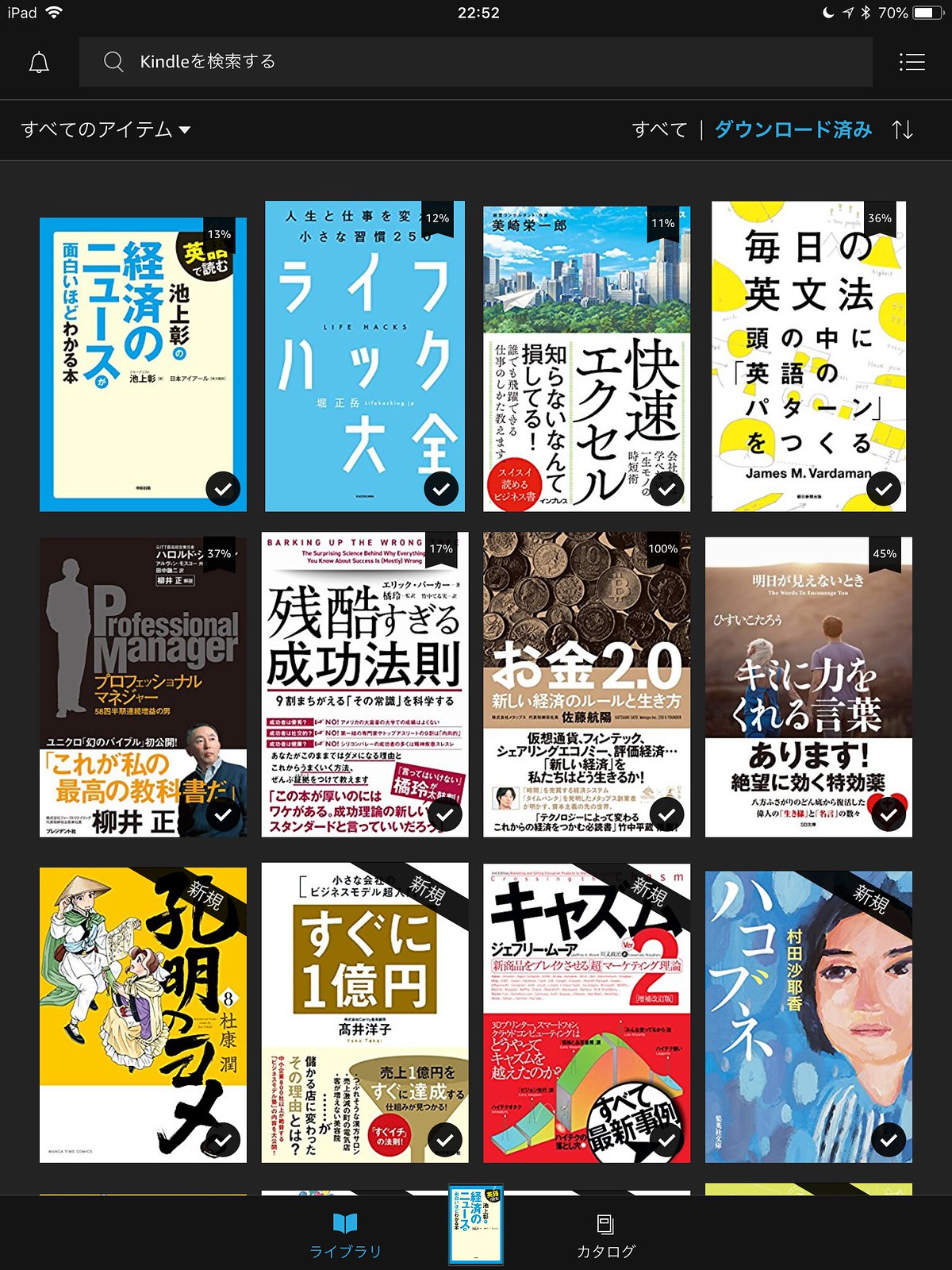This image is a screenshot from an iPad, evident from the Wi-Fi icon, the battery percentage at 70%, and the time displayed as 22:52 at the top of the screen. The browser window shows an address bar reading "Kindle" followed by some Asian characters, indicating that this is a Kindle webpage. The entire page is in an Asian language, possibly Japanese or Korean, featuring thumbnails of 12 different book covers or posters arranged in a grid with three rows of four items each. Each book cover includes a check mark in the bottom corner.

The book covers are diverse in color and imagery, with some notable details: a cover with coins on the front, one with a snow-capped mountain, another with a sandscape and a distant mountain, a cover featuring the silhouette of a man against a black background with gray text that resembles a movie poster, and one with an image of an Asian woman with dark hair and pale skin. The text on the covers is mostly in the Asian language, with the exception of one book that has "Professional Manager" written in English amidst the foreign text. The webpage has sections of white and blue Asian characters at the top, with a blue book icon and another icon resembling newspapers at the bottom of the screen. The book covers themselves are visually distinct with a variety of color schemes, including blue and white, white and yellow, and others.